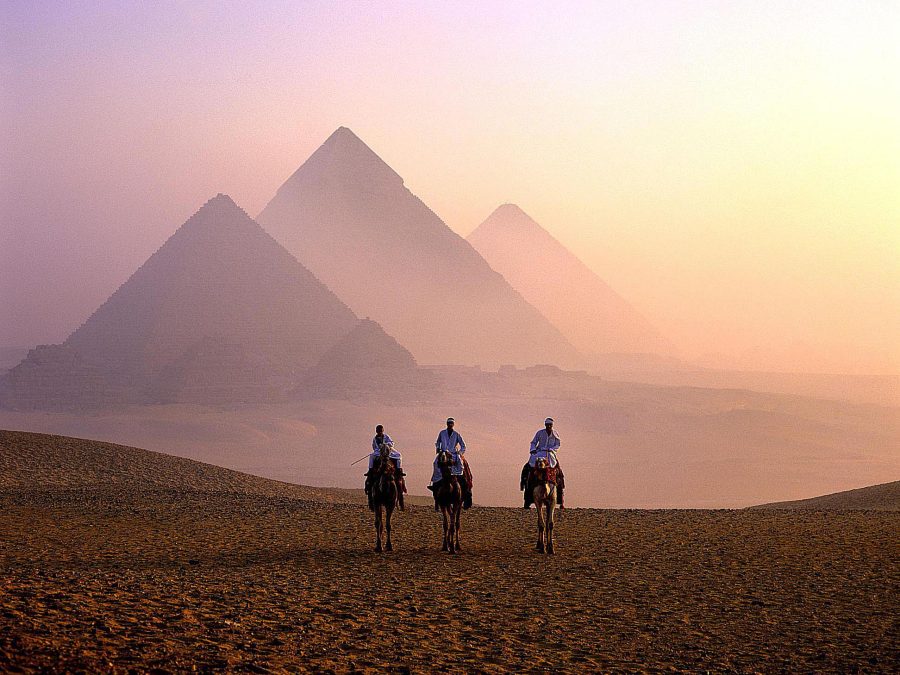In this captivating image, three men are shown riding camels through the vast, sandy desert near the Great Pyramids of Giza. Each man is dressed in a bluish-white robe and headband, sitting atop saddled camels that stand closely together. The desert ground beneath them is a sweeping expanse of tan sand. The backdrop reveals an impressive view of both the three iconic Great Pyramids of Giza and several smaller pyramids, their contours softened by a hazy, foggy atmosphere. The sky above is a gradient of pink, blue, and orange hues, suggesting either the early morning or the approach of sundown. The entire scene is devoid of any vegetation or buildings, emphasizing the unbroken desert landscape and the majesty of the ancient pyramids against a serene, color-streaked sky.